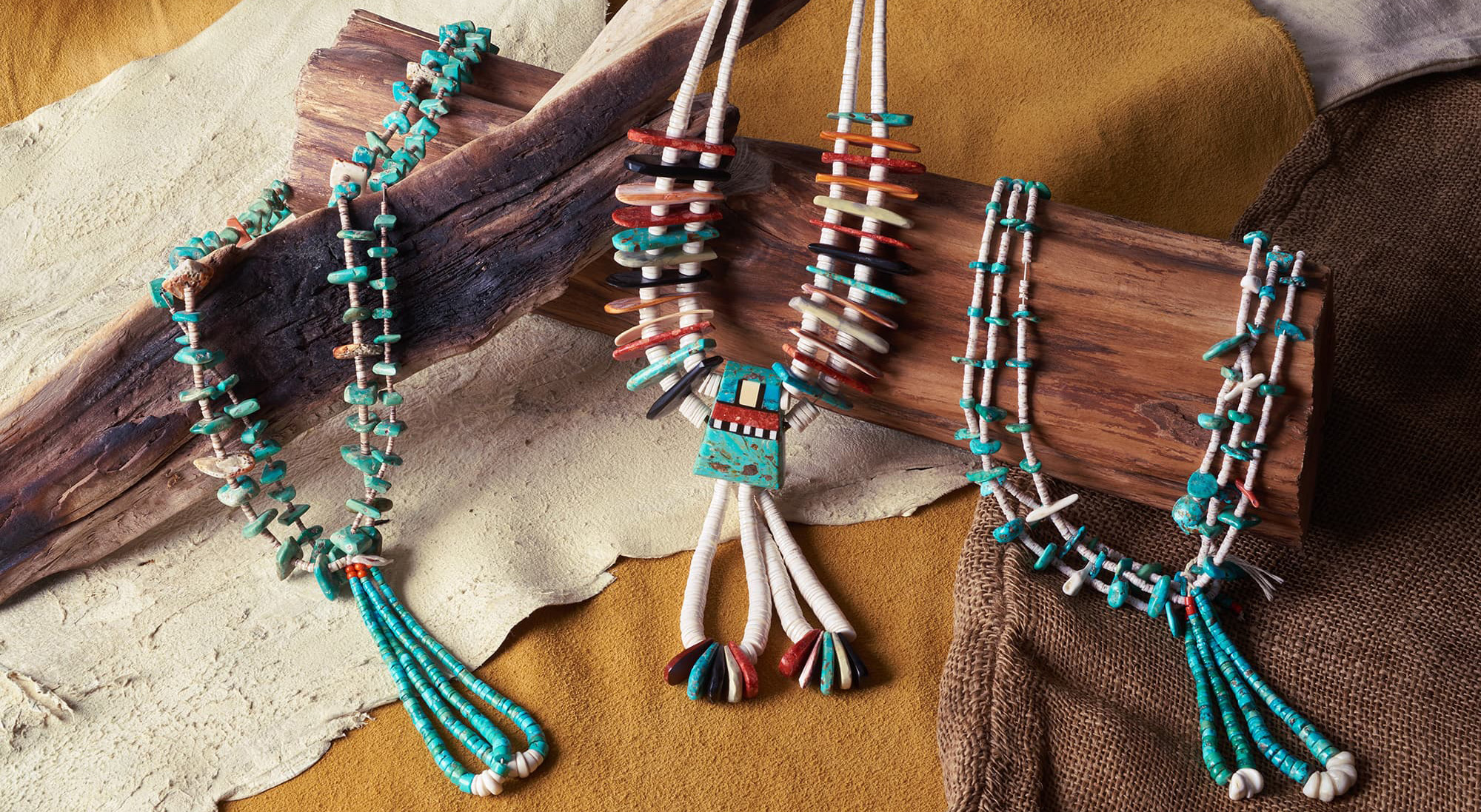The image displays three intricate Native American necklaces showcased on a rustic and natural background. The background is composed of white and brown pieces of hide arranged on a table, with two split logs positioned on top of the leather. The necklaces, crafted with great detail, are draped over these logs. Each necklace is a stunning example of Native American art, made primarily of turquoise beads with accents of red, black, and white. The beading is meticulous, covering the strings entirely, and each piece features its own unique pattern. The turquoise beads dominate the color scheme, with one necklace being mostly blue, another showcasing a mix of blue, white, and red, and the third combining blue and white hues. These beautiful, handmade necklaces exude a traditional yet timeless charm, highlighting the skill and artistry of their creators.